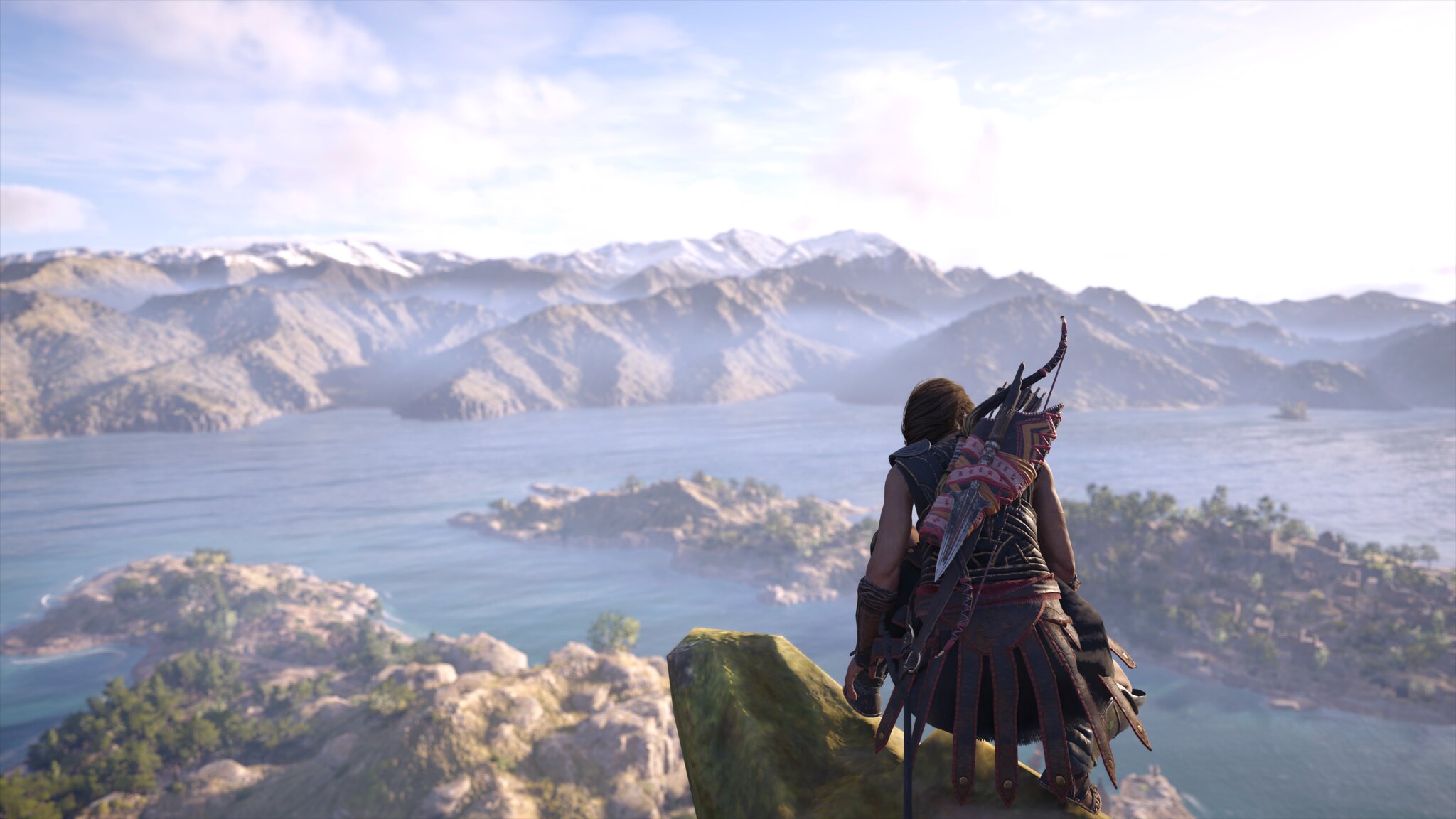In this hyper-realistic screenshot from a high-quality video game that might also be mistaken for an animated movie, a warrior stands prominently on a green rocky outcropping overlooking a vast, sunlit landscape. The warrior, seemingly a woman with dark brown hair, is adorned in leather armor and arm guards, with a bow and a quiver of arrows slung across her back. She kneels with her left leg forward, facing away from the camera. The scene is bathed in bright sunlight streaming from the top right corner, creating a desaturated environment around her, yet she remains distinctly more contrasted against the backdrop. The panoramic view reveals a vast ocean dotted with small islands, an expanse of land, and distant mountains—some of which are capped with snow—rendering a breathtaking, picturesque vista.